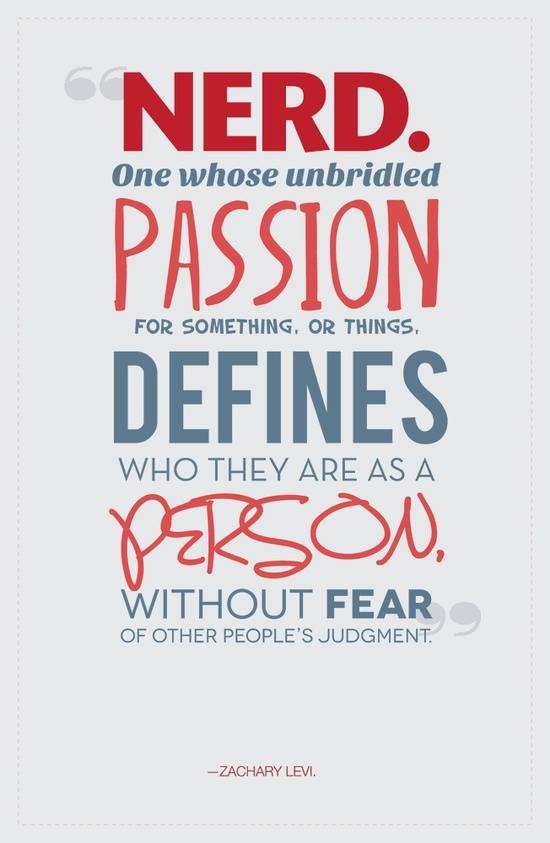The image features a quotation on a white background, with prominent centered text in various fonts and colors. At the top, there are gray quotation marks framing the text. In large, red, capitalized letters, it reads "NERD." Below that, in blue font with only the 'O' capitalized, it states, "One who's unbridled passion," followed by a lighter red, larger font for the word "PASSION." Continuing in smaller blue font, it says, "for something or things defines in," followed again by blue, "ALL CAPITAL LETTERS." The next line in thinner all-capital blue font reads, "who they are as a," and the subsequent line in a red, cursive-print combination states "PERSON." Lastly, it concludes in blue text, "without fear of other people's judgment," with the word "fear" in dark blue and the rest in lighter blue. At the bottom, in small red font, it is signed "Zachary Levi."